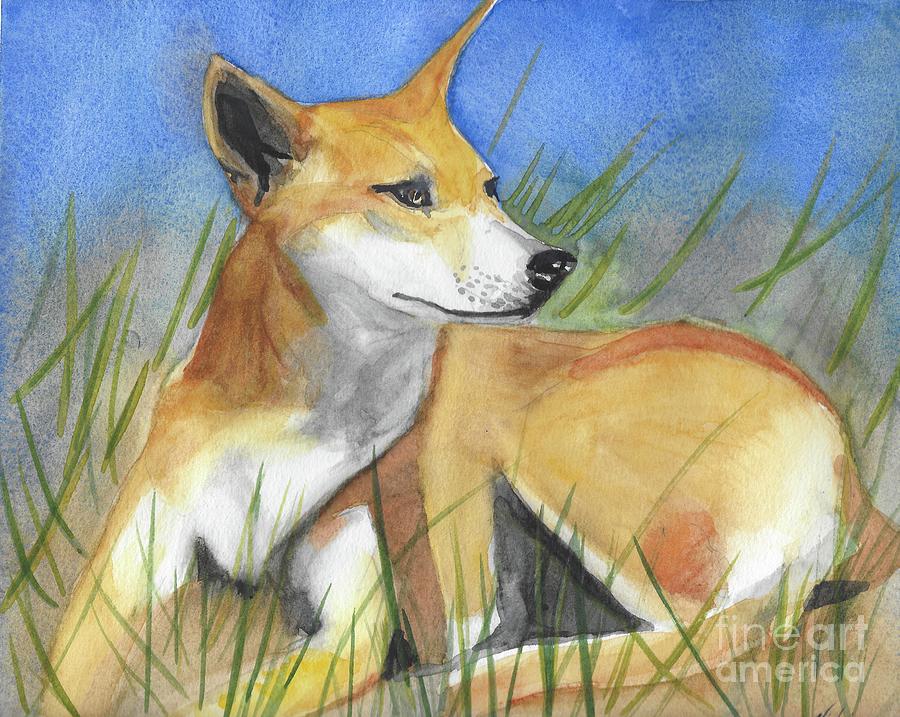In this detailed painting, a tan-colored dog with creamy, almost orangish fur detailed with white on its snout and underbelly, reminiscent of a dingo, sits alertly on thin, wispy grass that could be sea grass. The dog's body faces left while its head tilts to the right, ears perked and eyes keenly focused as if responding to a distant sound. The serene scene is set against a pale blue sky with subtle darker areas, adding depth to the backdrop. The bottom right corner of the painting bears the watermark of Fine Art America, confirming its artistic provenance.